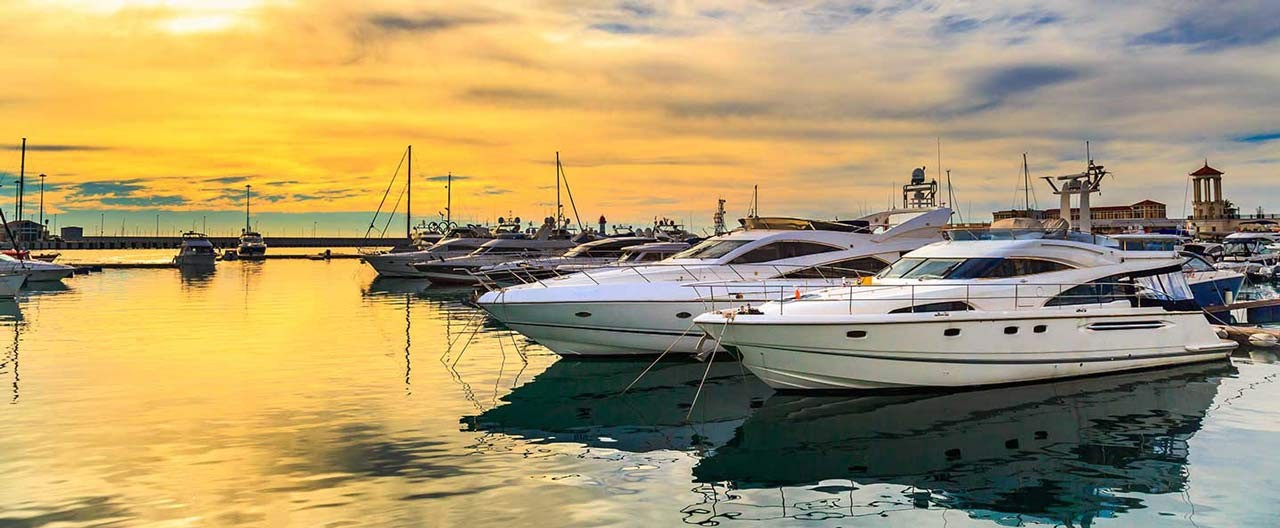The professionally-taken photograph captures a serene sunset scene at a marina. The sky is a stunning blend of white, yellow, blue, orange, and gray hues as the sun sets, casting a warm golden reflection on the tranquil blue waters. The marina is populated with 10 to 15 boats, primarily white with blue accents, all docked at their slips. These are private vessels, mainly used for sailing, and none are currently in motion. The boats are neatly backed into the pier with bow ropes extending to anchors, and in the background, a variety of building structures in black, white, gray, silver, brown, blue, yellow, and orange can be seen, including a distinct bell tower and a long, low building. There is a clear view of the waterway leading out to a larger bay, with a few ships visible on the horizon. Some people are walking along the far end of the pier, adding to the peaceful ambiance of the scene. There is no text in the image.